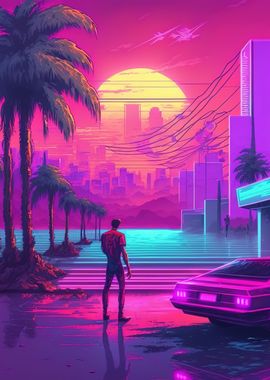This illustration depicts a man standing on a neon-hued ground, facing away from the viewer towards a distant cityscape bathed in vibrant colors. His muscular frame is clad in red clothing, and he stands beside a magenta-colored car on his right. The cityscape ahead, tinted in shades of purple and red, is silhouetted against a dramatic, hot pink sky with a large, semicircular yellow sun hanging low on the horizon. To his right, buildings rise against the sky, some adorned with visible power lines. On the left side, a row of green palm trees lines the walking path, adding a touch of natural greenery to the otherwise vividly colored scene. The entire scene is infused with intense, neon lights that create an atmospheric glow around the man and the environment.